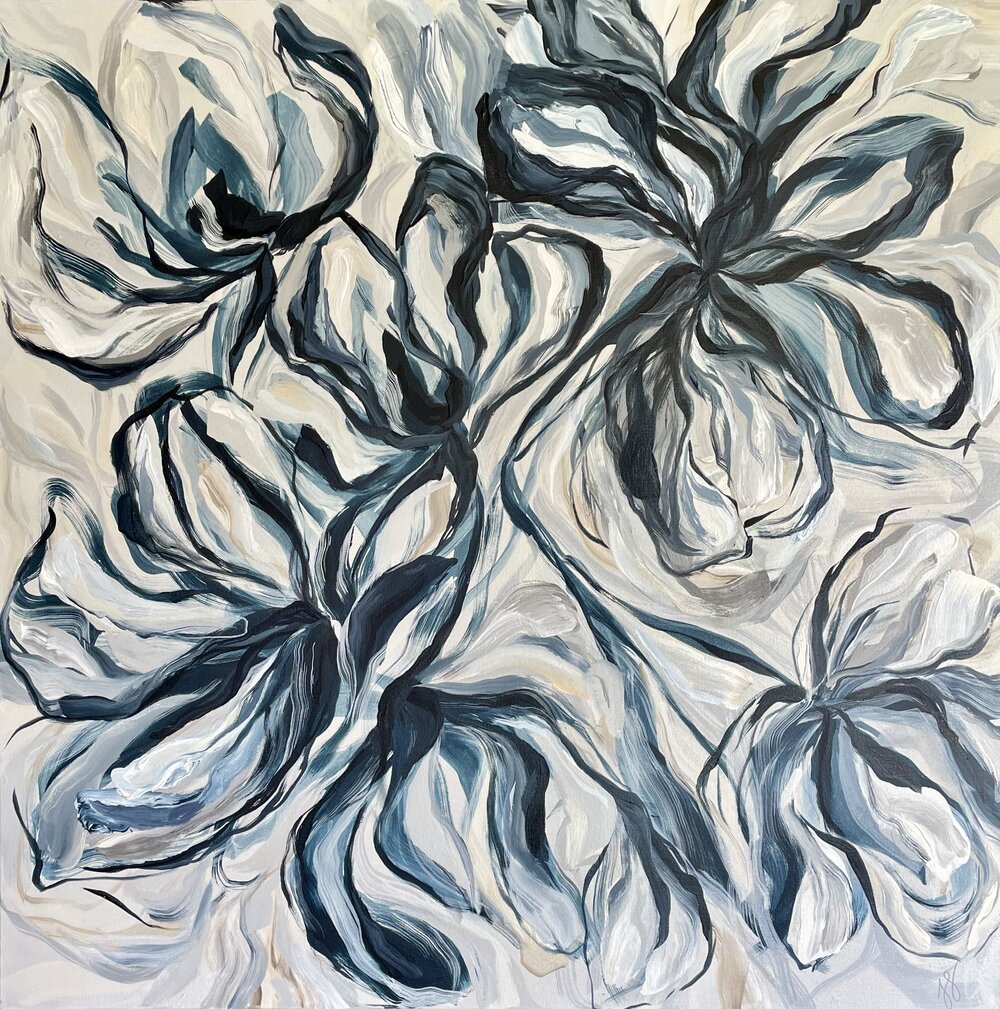The painting exhibits an intricate abstract representation of flowers, with an impressionistic style. Dominated by a range of colors including black, dark blue, white, gray, beige, and hints of light yellow, the canvas showcases a bouquet-like arrangement of about six flowers with varying formations of petals. The petals and stems meander in wavy, winding lines and curves, contributing to a nearly symmetrical yet chaotic harmony. The top right of the painting features a distinctive flower, while the top left possibly depicts a closed bud. More flowers, either open or closed, are distributed in the bottom right and bottom left. The brush strokes are spread evenly across the canvas, suggesting a balanced composition despite the abstract nature. In the top right corner, text that appears to be ‘JJ in person’ might indicate the artist's signature. The image seems to be captured indoors under controlled lighting, focusing solely on the painting without any visible frame or surroundings. The medium used could potentially be acrylic or watercolor, emphasizing the fluid and dynamic aesthetic of the floral arrangements.